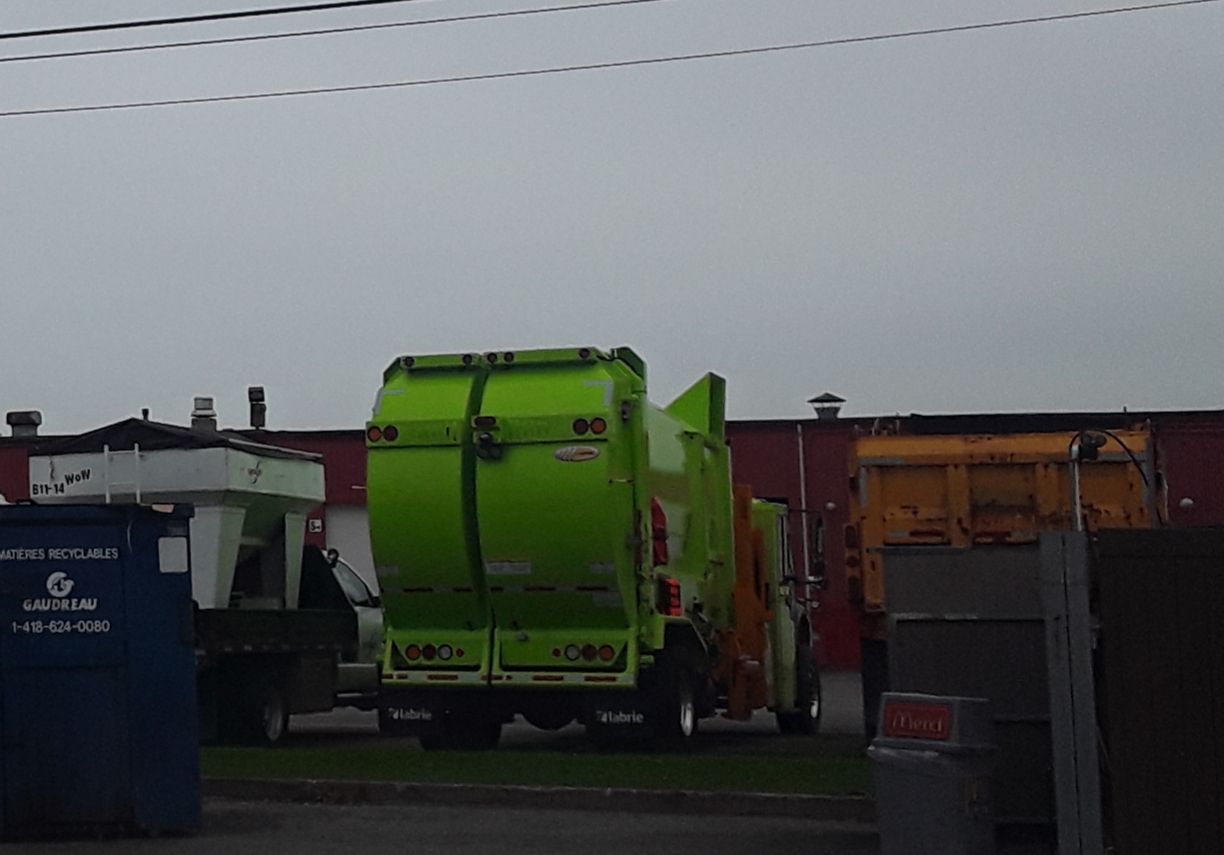In the photograph, there is a lime green garbage truck prominently featured, which appears to have dual disposal areas for regular trash and recyclables, as inferred from its divided rear. The scene is set on a dreary, overcast day, casting a grayish hue over everything. The green garbage truck is backed into a parking spot, flanked by a black truck with a white structure on its left and an older, orange dump truck on its right. In the foreground, there is a blue recycling dumpster marked with a phone number and a McDonald's trash can labeled "Mercy" with the iconic golden arches. The background showcases a long red wall, which could be part of a building or a fence, adding to the industrial feel of the setting. Gray dumpsters can also be seen on the right. Overall, the scene appears to be a worksite, with the trucks parked and ready for action against a gloomy backdrop.